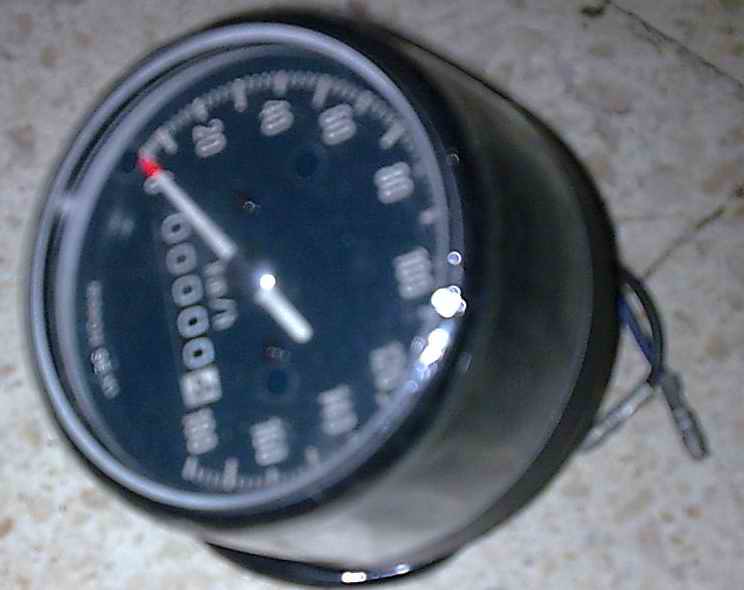The image captures a black cylindrical gauge, positioned horizontally on a tiled stone floor. The gauge features a black exterior covering and a series of numerical markings ranging from 0 to 120, though the image becomes blurry beyond those points. A white needle with a red tip is centered at the zero mark. Below the needle, there is a numeric counter displaying '00000'. Additional writing is present at the bottom of the gauge's face. In the background, a wire can be seen hanging behind the gauge. The stone tile flooring is composed of white and light yellow colors, resembling tiny pebbles interspersed within the tile.